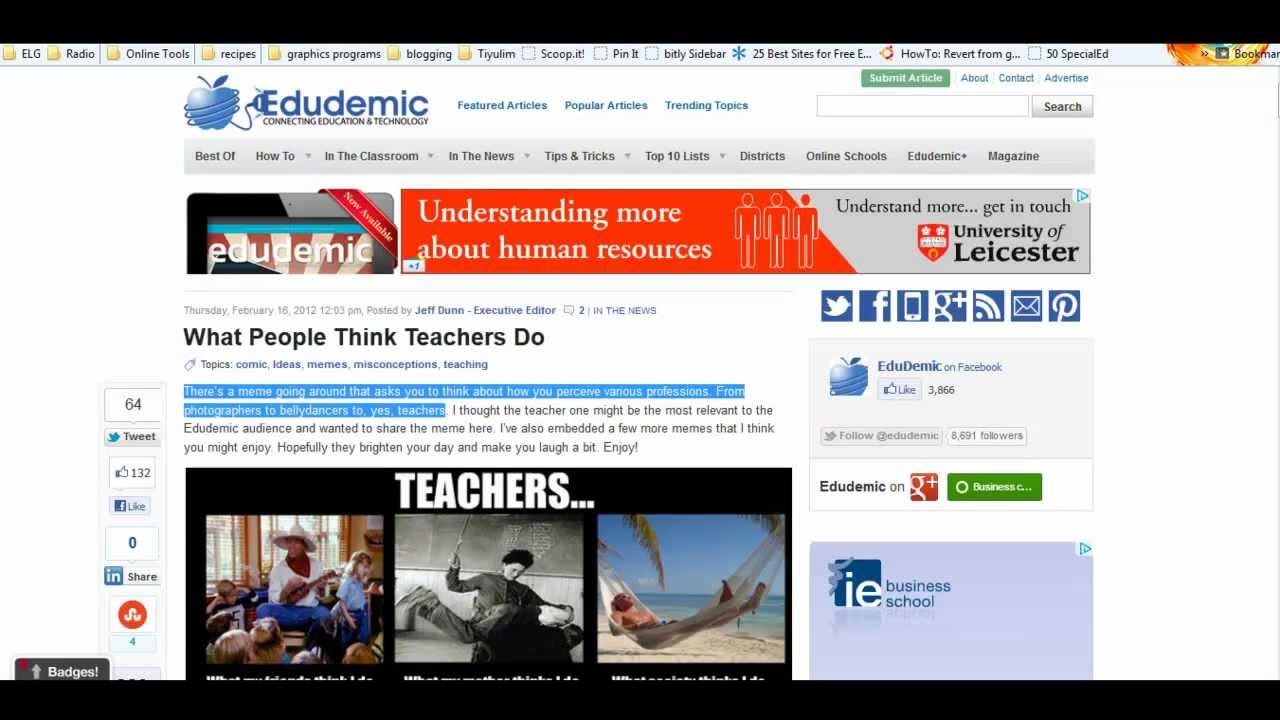A screenshot depicts a website featuring a predominantly red, blue, black, and white color scheme. In the upper left corner, there's a white frame that contains an illustrated logo. The logo showcases a blue apple entangled in a matching blue cord, with the cord's end stylishly plugging into the word "edudemic," also rendered in blue. Directly beneath this logo, a detailed navigation menu is visible, listing various options: "Best Of," "How To," "In The Classroom," "In The News," "Tips and Tricks," "Top 10 List," "Districts," "Online Schools," "Edudemic," and "Magazine."

Just below the navigation bar, a prominent red banner spans the width of the page, with the slogan "Understanding More About Human Resources" inscribed in bold white letters. Further down, a black headline reads "What People Think Teachers Do," introducing the beginning of an article accompanied by additional images that suggest further content related to education and human resources.